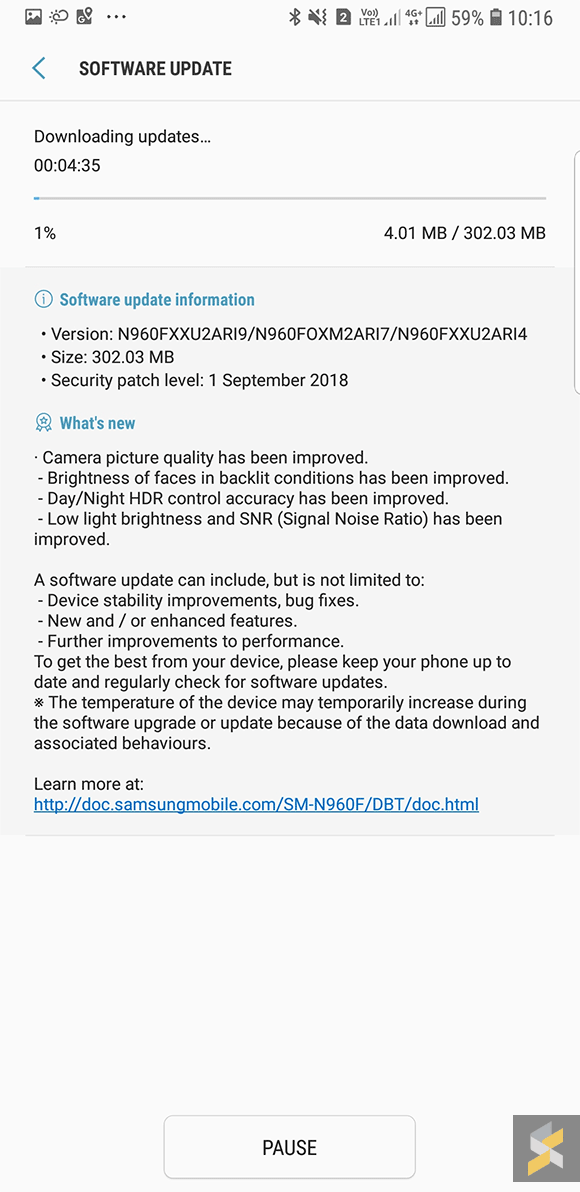This image depicts a software update screen on a mobile device. The software update is currently in progress, having downloaded 1%, which equates to 4.01 MB out of a total 302.03 MB. Key details provided include:

- **Software Update Version:** Information not specified in the caption but mentioned.
- **File Size:** 302.03 MB.
- **Security Patch Level:** September 1, 2018.

The update notes highlight several improvements, particularly in camera functionality:
- **Enhanced Camera Picture Quality**
- **Improved Brightness of Faces in Backlit Conditions**
- **Refined Day and Night HDR Control**
- **Optimized Low Light Brightness and Signal-to-Noise Ratio (SNR)**

Additional improvements include:
- **Device Stability Enhancements**
- **New and Enhanced Features**
- **Overall Performance Improvements**

The screen also emphasizes the importance of keeping the phone up to date for optimal performance and security.